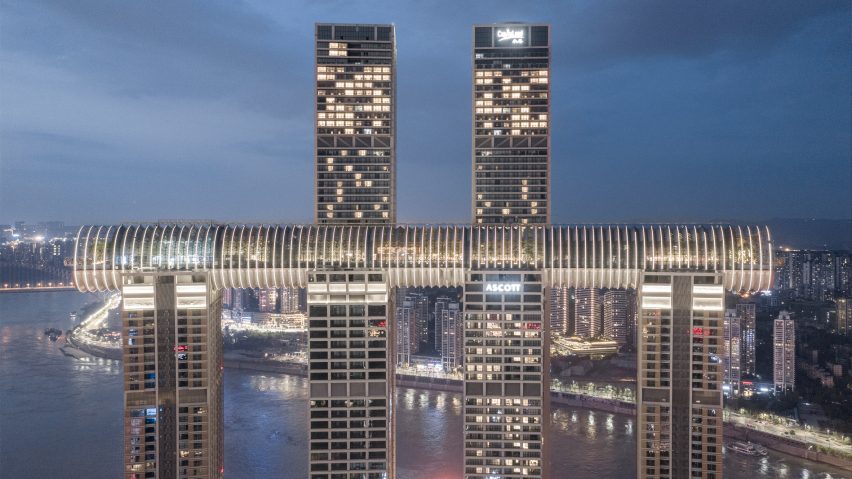This captivating nighttime photograph features an intricate cityscape along a waterfront. At the core of the image, four prominently silver and white high-rise structures stand evenly spaced in sequence from left to right. These buildings are interconnected by a large, tubular structure that stretches horizontally across their tops. The tube is particularly striking, as it is transparent and encircled with thin, evenly spaced gold rings. On top of this cylindrical structure, two taller, rectangular skyscrapers ascend, mirroring each other in height and dominating the skyline. The skyscrapers feature illuminated windows, adding vibrancy to the scene, particularly in the third building from the left which brandishes the glowing text "ASCOTT."

The background reveals a bustling city bathed in light against a dark blue night sky, with reflections shimmering off a waterway that lines the edge of the urban landscape. The overall scene is a blend of architectural beauty and illuminated grandeur, capturing the essence of a thriving metropolis at night.